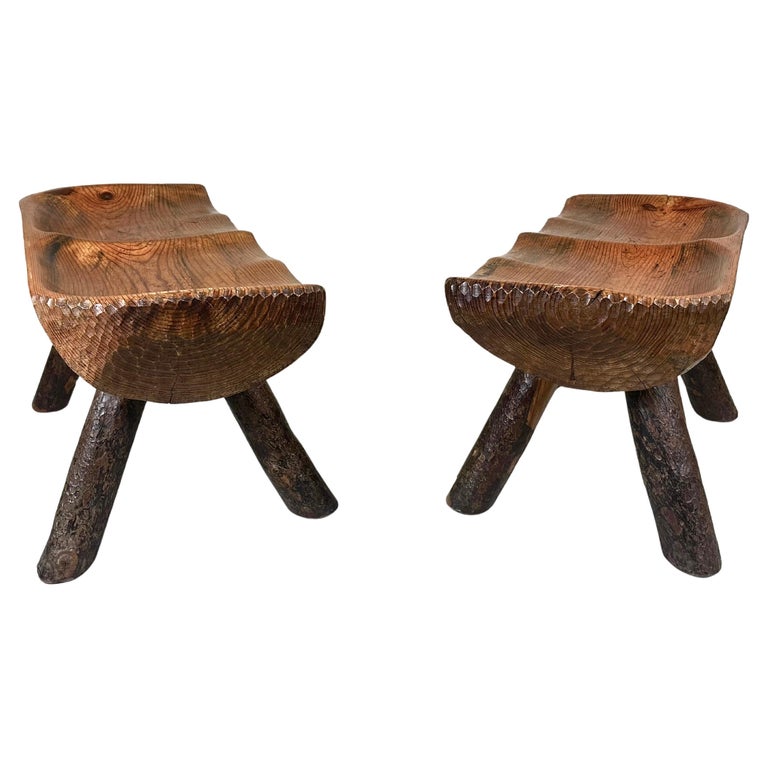The image showcases two identical handcrafted wooden benches, each appearing as double-seated stools with natural, rounded shapes. The benches are made from large tree trunks, smoothly split in half to form ergonomic seats with subtle, comfortable indentations for sitting. The fine craftsmanship is evident in the careful whittling and carving, which retains the texture and grain patterns of the original wood. Each bench is supported by four sturdy, branch-like legs that enhance their rustic yet finished appearance. Positioned facing each other diagonally, the benches stand on a completely white background, which highlights their brown hue and intricate details, including the circular grain on the sides and potential tribal-inspired carvings that add to their unique charm. Overall, they exude a sense of robust durability and aesthetic beauty.